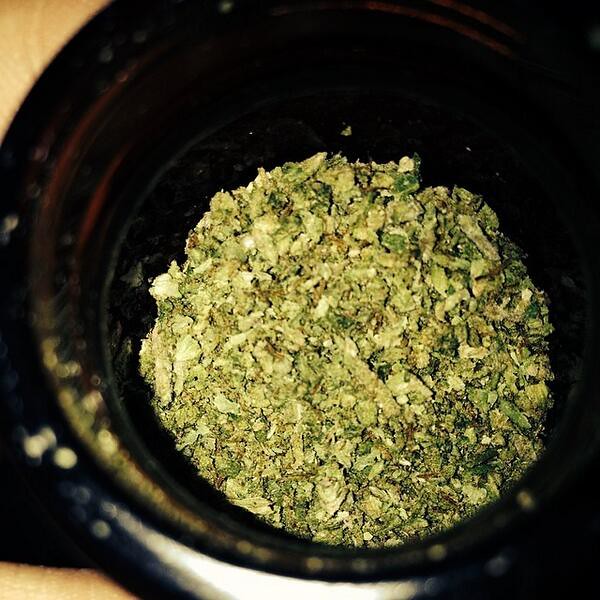In the photograph, a black, ridged bowl with a narrow base and wider top sits on a light tan countertop. The black bowl, which could be plastic or glass, contains a mixture of fine, ground-up green substances—perhaps marijuana, dehydrated broccoli, or another dried green vegetable. The green particles are interspersed with small brown and darker brown pieces resembling grains or chopped vegetables, resembling dirt in texture and appearance. This dry mix predominantly covers the bottom of the bowl. The image, taken from a vertical perspective, also shows glimpses of the wooden table or countertop at the photograph's top and bottom corners.